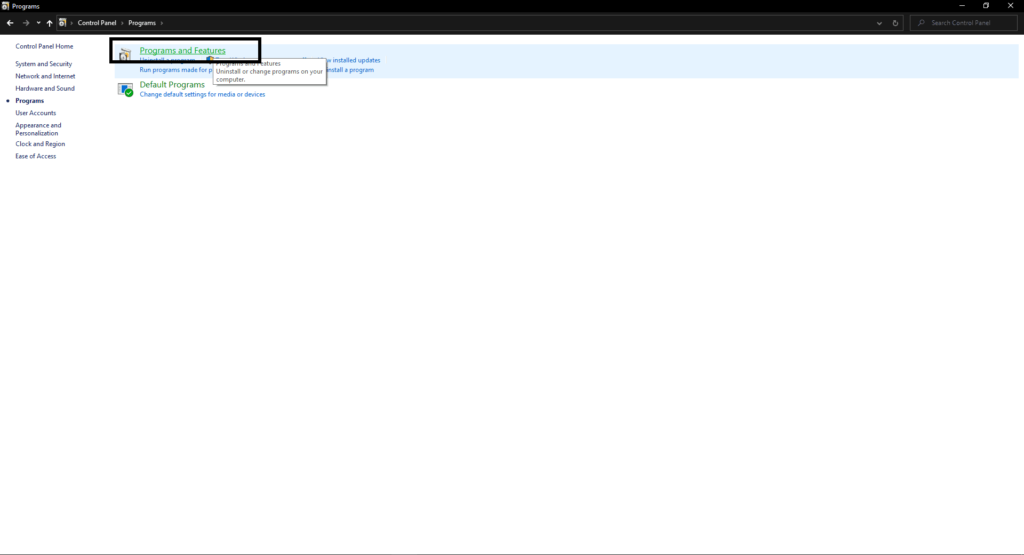The image is a screenshot of a web page displaying the control panel of a Windows computer. The top section features a dark black bezel, where the term "Programs" is written next to an icon resembling an open box with a clock, possibly representing the "Programs and Features" section. To the left, a bold white arrow suggests the option to navigate back, while a grayed-out forward arrow indicates that no forward progress has been made yet. A white dropdown arrow and an upward arrow are also visible in the bezel.

On the right-hand side, the same icon of a box and a disk is repeated, accompanied by an arrow pointing to the right, which directs to subfolders within the control panel. The "Programs and Features" section is selected and highlighted by a black rectangle around it. The heading "Programs and Features" is presented in green hyperlink text, with additional blue hyperlink text beneath it, although the latter is partially obscured by two overlapping rectangles. The second rectangle is a Windows pop-up with black text on a white background, explaining "Programs and Features" as a section to uninstall or change programs on the computer.

Below this pop-up, there is a gray box with tiny black text, a small blue box, and a green circle featuring a white checkmark. This section pertains to "Default Programs" highlighted in green hyperlink text, with blue hyperlink text below it stating, "Change default settings for media or devices."

On the left-hand side, the control panel navigation menu is visible with dark blue text. The menu items listed are:
- Control Panel Home
- Systems and Security
- Network and Internet
- Hardware and Sound
- Programs (boldened with a circle next to it indicating it is selected)
- User Accounts
- Appearance and Personalization
- Clock and Region
- Ease of Access